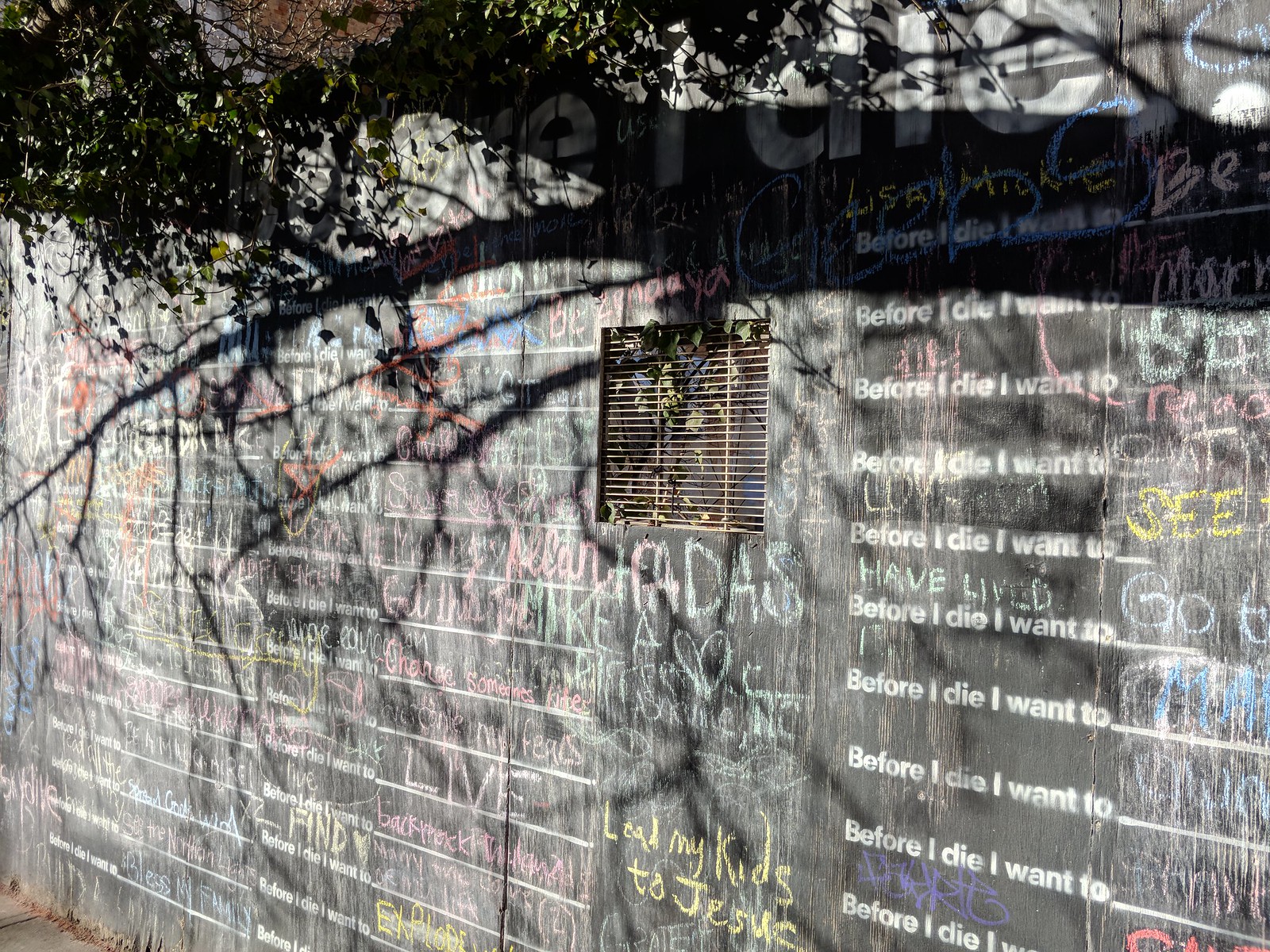This photograph depicts the side of a club that has been transformed into a large blackboard wall covered in colorful chalk writing and drawings in hues such as yellow, green, blue, white, and pink. The wall features a small square window, either barred or with blinds, and is partially shaded by the overhanging branches of a large green tree. The central theme of the chalkboard is "Before I die I want to…," with spaces for visitors to fill in their wishes and dreams. Areas of the wall are difficult to read due to the sheer number of inscriptions, but notable entries include "Before I die I want to explore something" and the poignant "Before I die I want to live." The black shadow cast by the tree adds depth to the poignant scene, making the wall a dynamic, ever-changing canvas of collective aspirations and artistic expression.